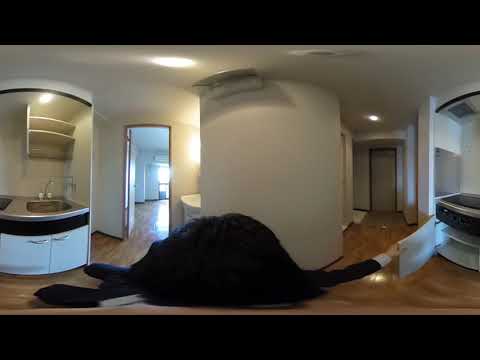The image showcases a panoramic view of a minimalist, modern kitchen inside an apartment or house. The floor features medium brown wooden planks that complement the white walls and cabinetry throughout the space. The central figure, distorted by the 360-degree camera effect, appears with an exaggerated head and smaller body parts, particularly noticeable as they open a cupboard beneath a black stovetop without an oven, nestled within white cabinets on the right. The stovetop features dials and control panels with an air vent overhead. To the left of the figure is a stainless steel sink with white cabinets below and shelving above, marked by horizontal silver handles and a small, bright light fixture. Open doorways show glimpses into other rooms, allowing natural sunlight to flood in and reflect off the wooden floor. The scene hints at a property showing, given the absence of personal items, making it appear staged for sale. The walls and ceiling in the center are curved, housing a rectangular air conditioner unit close to the ceiling. A corridor visible on the right leads to another closed door further accentuating the streamlined, clean design of the space.